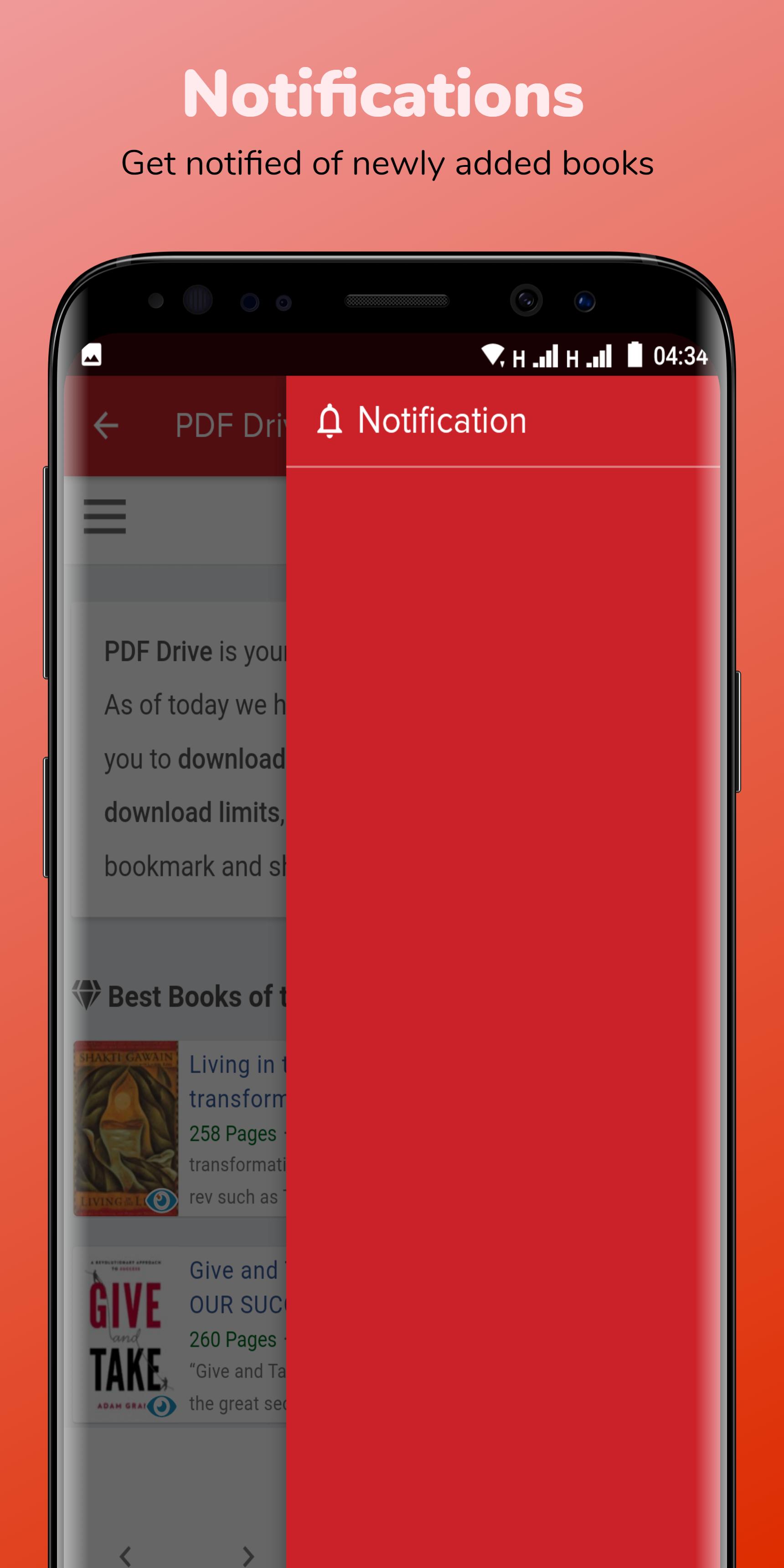The image features a smartphone set against a gradient background, transitioning from peach at the top to a deeper orange at the bottom. On the screen, the notification panel is prominently displayed with a white header reading "Notifications" and a black subheading that states "Get notified of newly added books." The phone interface shows standard icons at the top like Wi-Fi, signal bars, and the time, which is 4:34.

A red notification bar extends from the right edge of the screen, covering roughly two-thirds of it. At the top of this bar, another "Notifications" label is shown, accompanied by a bell icon. Below, there's a blank line, followed by white text indicating app content, including truncated text like "PDF," "PDF Drive is your," and partially visible phrases related to downloads, bookmarks, and book titles, all incomplete due to screen cutoff. Specific phrases seen include "258 pages" and "give and take," associated with various book references, most incompletely displayed.